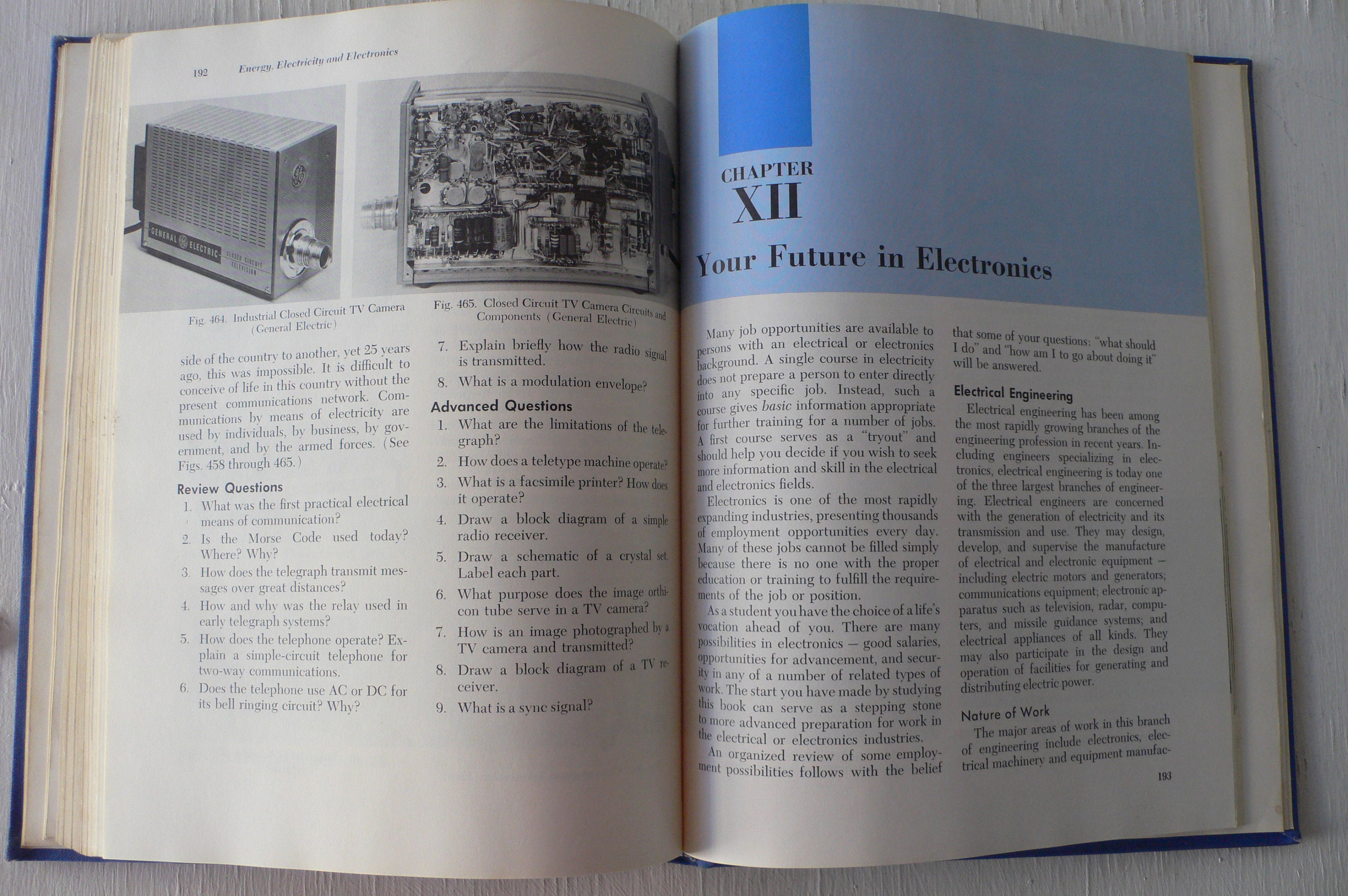The image depicts a large, well-worn textbook with a blue cover, open to pages 192 and 193. Page 192 introduces the topic of "Energy, Electricity, and Electronics" and features two images. Figure 464 is labeled as an industrial closed-circuit TV camera, while Figure 465 illustrates the circuits and components of this TV camera. Beneath these images are review and advanced questions, suggesting that this page is the conclusion of a chapter. Meanwhile, page 193 begins Chapter XII, titled "Your Future in Electronics," and delves into the field of electrical engineering and the nature of the work involved. The textbook appears to be a reminiscent artifact, possibly from a high school, giving a sense of nostalgia.